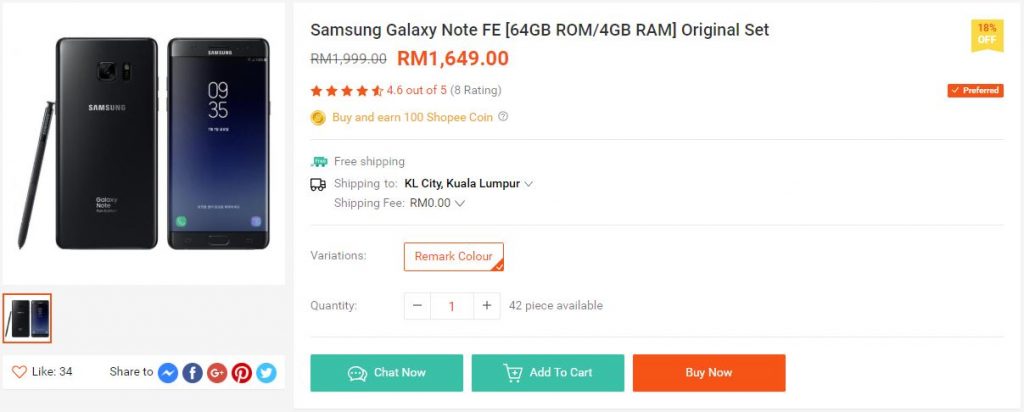The image depicts a shopping interface for purchasing a Samsung Galaxy Note FE smartphone. On the left side, there are front and back views of the Samsung Galaxy Note FE. The right side provides detailed product information, including specifications noting "64GB ROM / 4GB RAM" and indicating it is an "Original Set."

The original price listed was RM 1,999.00, now discounted to RM 1,649.00, marked with "18% off" in the upper right corner on a ribbon label. The product has a rating of 4.6 out of 5 stars based on 8 reviews. Additionally, buyers can earn 100 Shopee coins with this purchase.

There is a gray line separating the product details from shipping information, which mentions free shipping to Kuala Lumpur (KL City). There is an option for free shipping marked as "RM 0.00" with a pull-down menu. Under "Variations," the color is highlighted in a white box with a red outline and font.

"Quantity: 1" shows there are 42 pieces available for purchase. The interface includes interactive buttons: "Chat Now" in a green box with white text, "Add to Cart" in green with white text, and "Buy Now" in red with white text. The listing is also marked as "Preferred" in a blue and orange rectangle, indicating a trusted seller status.